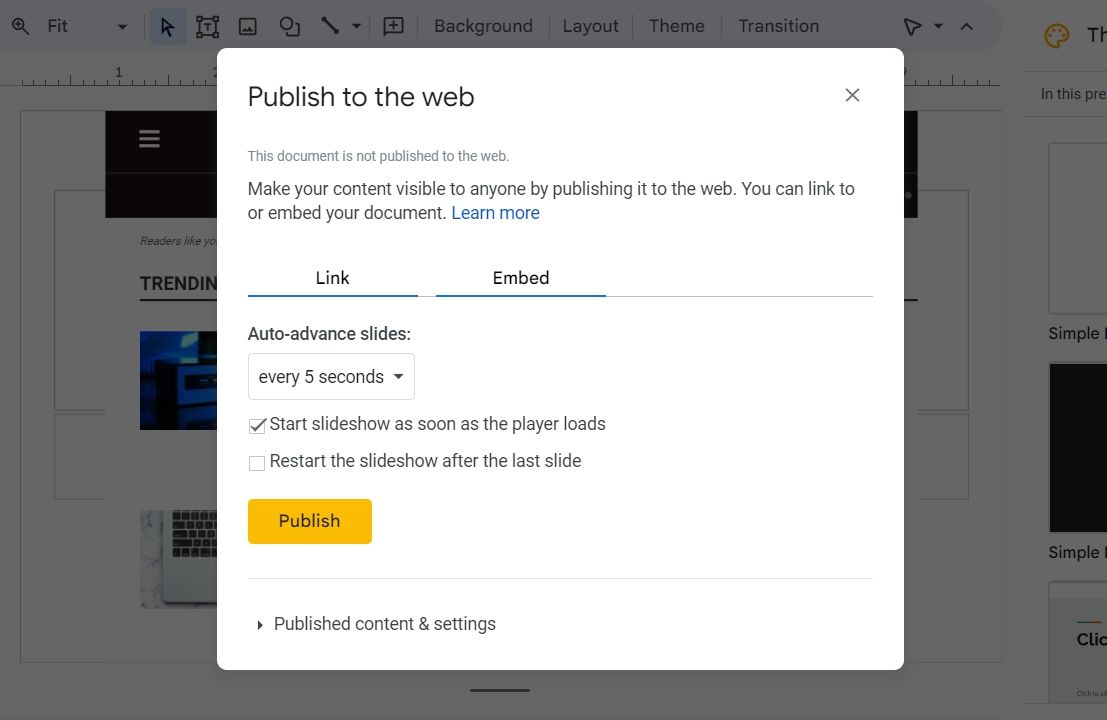A user is working within Google Slides, and a splash screen for "Publish to the web" is prominently displayed. This screen provides options to make the presentation accessible online, allowing viewers to link to or embed the document. Instructions are shown for setting auto-advance slides, currently set to every five seconds, with checkboxes for starting the slideshow as soon as the player loads (checked) and restarting the slideshow after the last slide (unchecked). A publish button is visible, indicating that the presentation is nearly ready for distribution. In the background, a partially visible image of a laptop can be seen, alongside a light gray interface. The slide pane on the right shows previews of individual slides, complemented by toolbar subsections like background, layout, theme, and transition. The main content of the presentation remains mostly obscured by the splash screen.